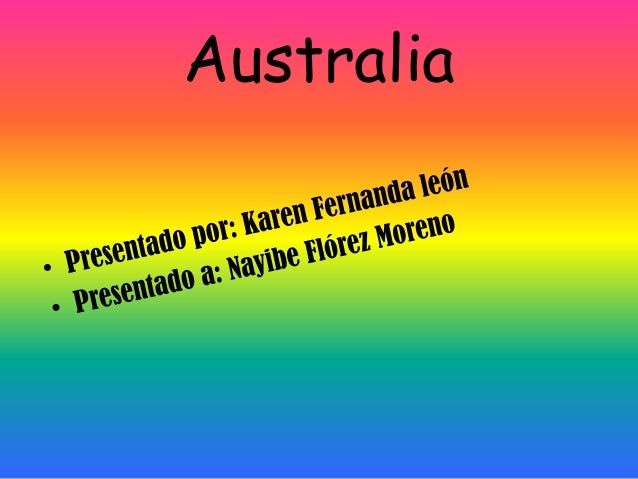The image appears to be a digital slide, possibly for a PowerPoint presentation, with a vibrant, linear gradient background transitioning from pink at the top, through red, yellow, green, and into blue at the bottom. At the top of the horizontal slide, there is a bold heading in black Comic Sans font that reads "Australia." Below this heading, there are two pieces of black diagonal text in a different font, positioned across the center of the image. The first line reads "Presentado por Karen Fernanda Leon," and the second line states "Presentado a Nayibi Flores Moreno." The entire composition features a vivid array of rainbow colors, and the text stands out clearly in black, suggesting a professional yet artistic presentation slide possible for a travel-related or educational context.